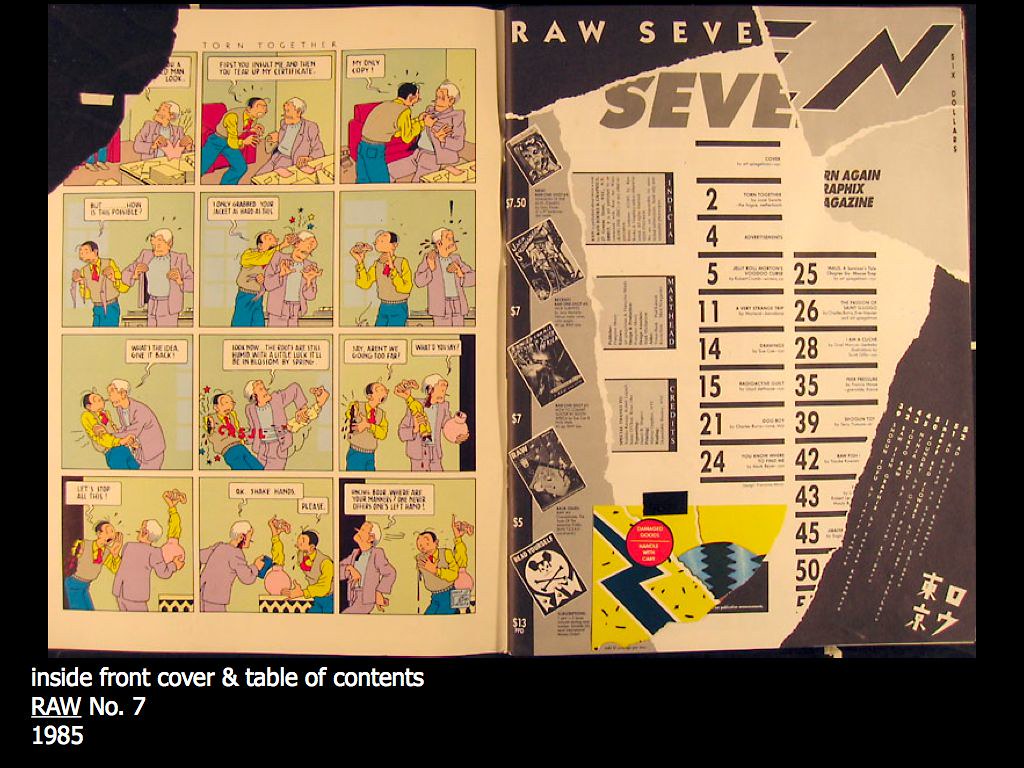The photograph depicts an opened comic book titled RAW number 7 from 1985, with the cover partially torn off, revealing only the upper-left corner. The comic is laid out facing down, displaying a two-page spread. On the left page is a comic strip featuring two men in a violent scene rendered in blue, light olive green, and purple hues, in which the text "torn together" is visible. The right page appears to function as a table of contents listing various page numbers (2, 4, 5, 11, 14, etc.) and includes some Japanese text, possibly indicating an international publication or translation. At the bottom of the image, on a black background with white text, it reads: "Inside front cover and table of contents, RAW number 7, 1985."